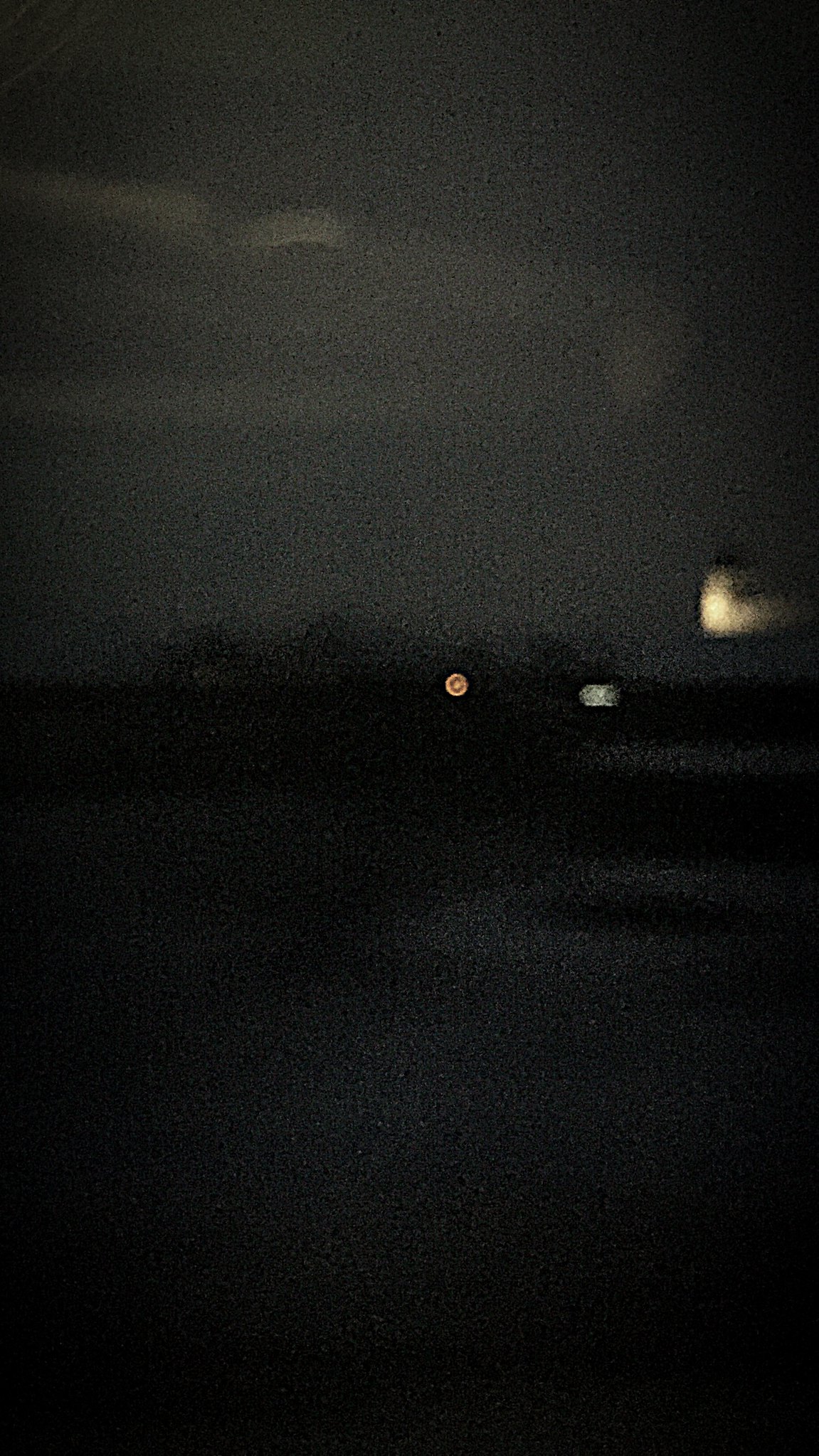This photograph, likely taken outside at night, is dominated by shades of gray and black, with subtle details in yellow. The image appears grainy, possibly due to a high ISO setting on the camera, leading to a noticeable dotting effect, especially in the darker areas. The sky is a mix of lighter grays, featuring cream-greyish streaks that might be clouds, giving it a slightly swirled appearance. Central to the composition is a bright yellow, or orange-ish, circle, which could be a distant light source from a house or car, casting minimal illumination. To the right, a small silver square can be seen, and above this is another yellowish, almost heart-shaped spot. The bottom half of the picture is significantly darker, with a prominent dark streak directly beneath the yellow circle, leading down to an even darker foreground.